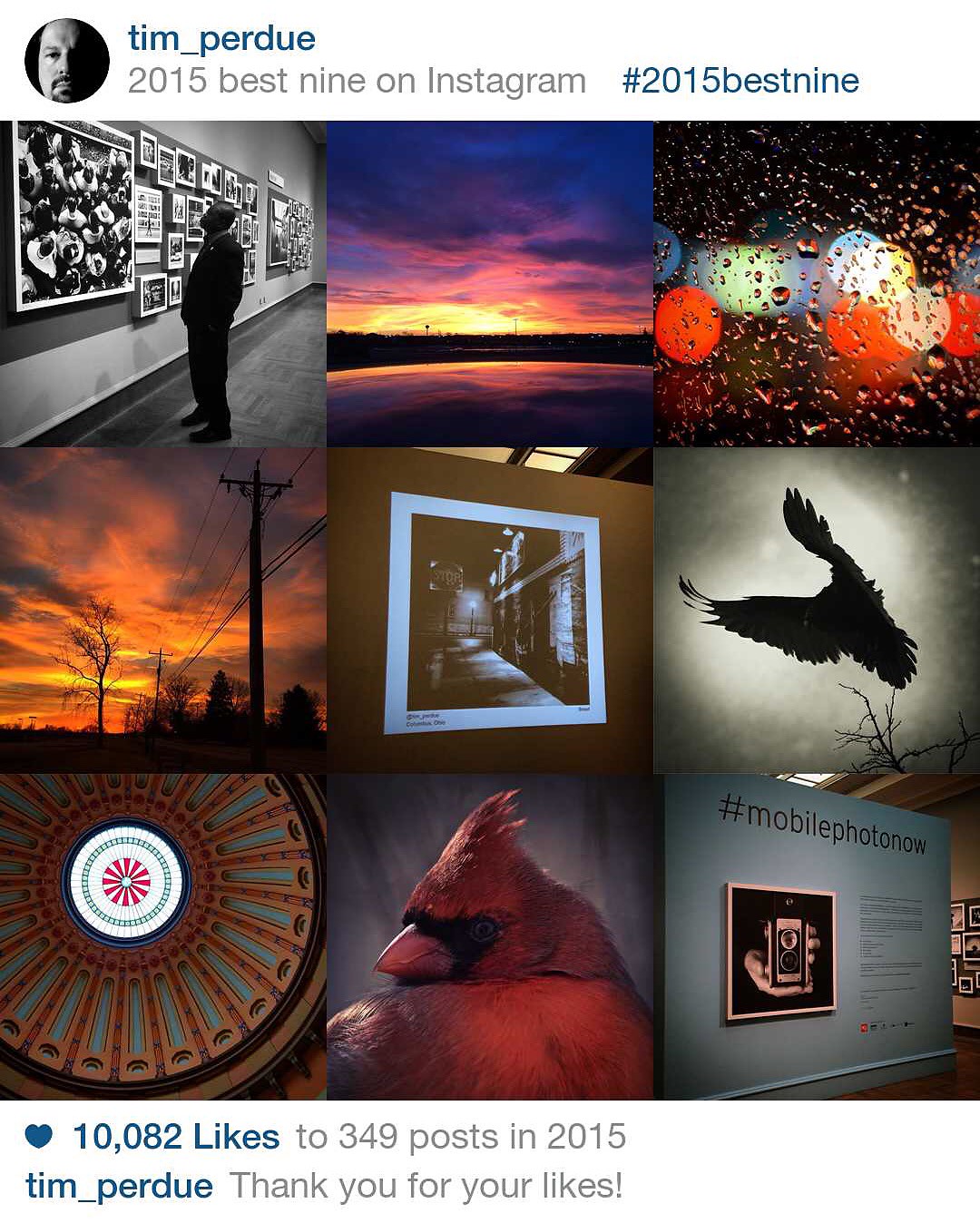This image is a collection of nine square-shaped photographs organized in a 3x3 grid format, visually presented as a highlight post from Tim Perdue's Instagram profile. At the top of the image, there is a small circular profile picture of a man beside the name 'Tim_Perude' in clickable blue text, followed by the heading "2015 Best Nine on Instagram" and the hashtag "#2015BestNine" in blue. 

The compilation includes a mix of different themes: 

- The first image is a black-and-white photo of a man looking to the left.
- The second image captures a colorful landscape sunset.
- The third image shows a cityscape during a rainy night, depicted through a windshield.
- The fourth is another breathtaking sunset over a horizon filled with trees.
- The fifth is another black-and-white photograph, although the subject is unclear.
- The sixth is a detailed close-up of a bird, specifically a cardinal.
- The seventh image portrays a cityscape, possibly the top of a building.
- The eighth image is another black-and-white photo, likely of a bird.
- The ninth and final image displays a museum exhibit with the hashtag "#MobilePhotoNow" and an image of a camera.

At the bottom of the collage, there is a blue heart icon indicating 10,082 likes and gray text mentioning that Tim Perdue made 2,349 posts in 2015. Beneath, Tim_Perude comments in blue text, "Thank you for your likes." The variety within these nine images highlights Tim Perdue's diverse photography skills, encompassing nature, urban settings, and creative compositions.